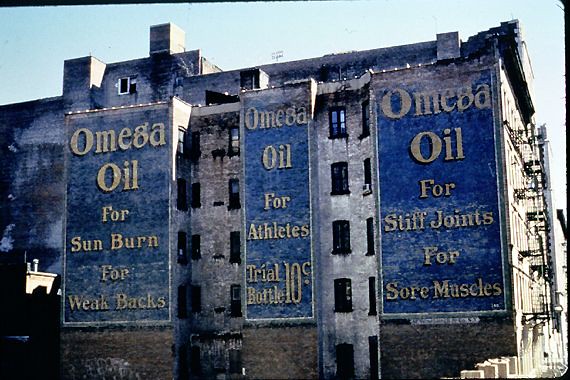The image depicts a large, old building, likely a factory or apartment building, featuring three prominent advertisements, each with a blue background and yellow writing. The first advertisement on the left reads "Omega Oil for sunburn for weak backs." The middle, thinner advertisement states "Omega Oil for athletes. Trial bottle, 10 cents." The right-most, thicker advertisement says "Omega Oil for stiff joints for sore muscles." The building is grayish with black windows, and looks weathered and dirty at the bottom of the signs, indicating age. Metal balconies or a fire escape can be seen on the right side of the building, contributing to its older architectural style. At the top, there's a structure resembling a chimney. The scene is set during daylight, with a blue sky visible in the background.